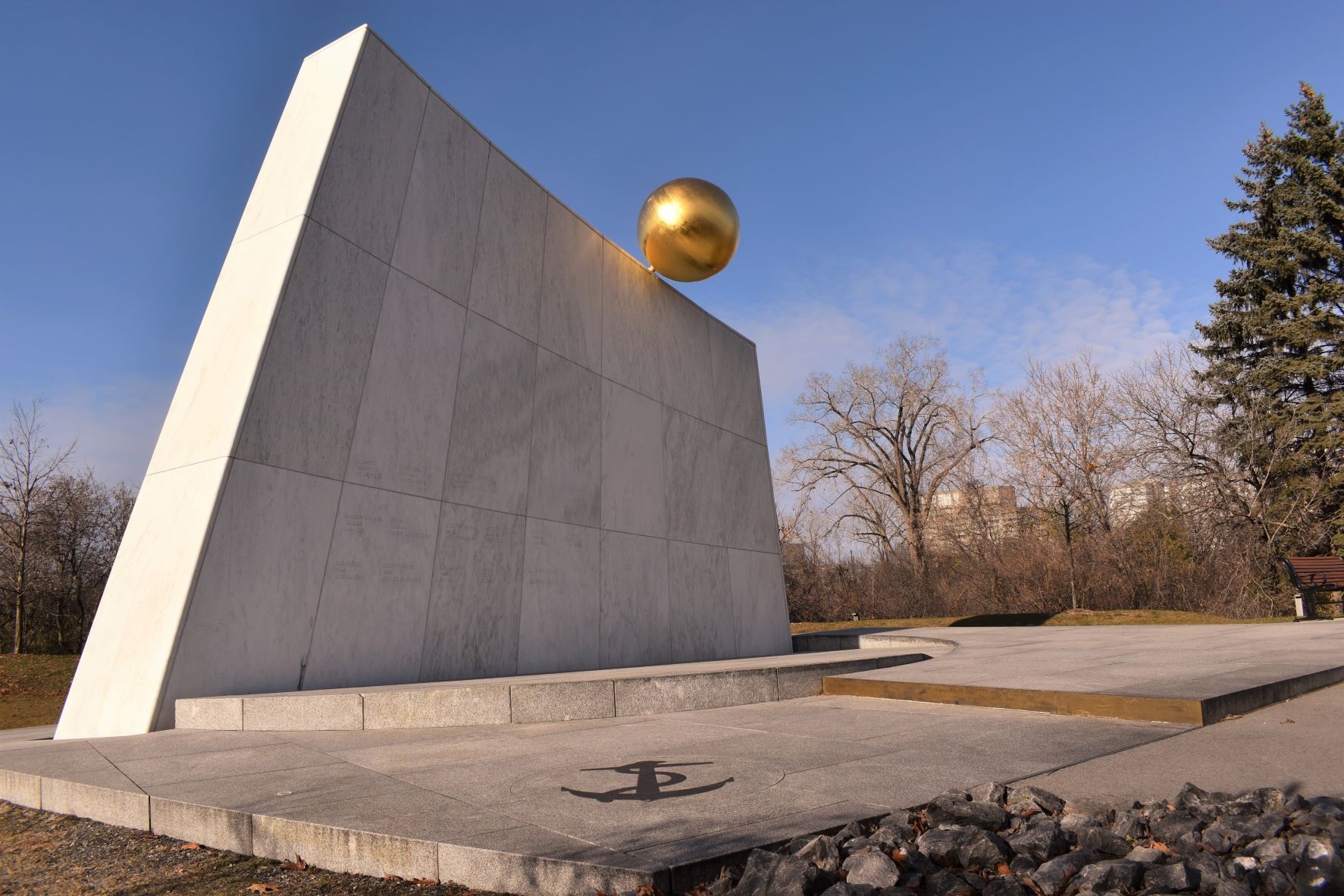The image depicts an outdoor monument characterized by a multi-leveled, modern structure. The centerpiece is a large, light gray concrete wall comprising 21 rectangular slabs stacked in three horizontal rows. At the top right corner of the wall, a striking gold metallic orb catches the eye. In front of this wall is a substantial concrete base, approximately six inches tall, featuring a black anchor symbol positioned at an angle in its bottom left corner. The base steps up to a higher level which gently curves around to the right. The surrounding scenery includes a field with large, leafless trees, suggesting it may be autumn or early spring. A blue sky with scattered white clouds forms the backdrop, and a tall pine or fir tree stands to the right, partially framed by a distant city skyline. Black gravel covers the ground at the monument's right side, completing the scene.